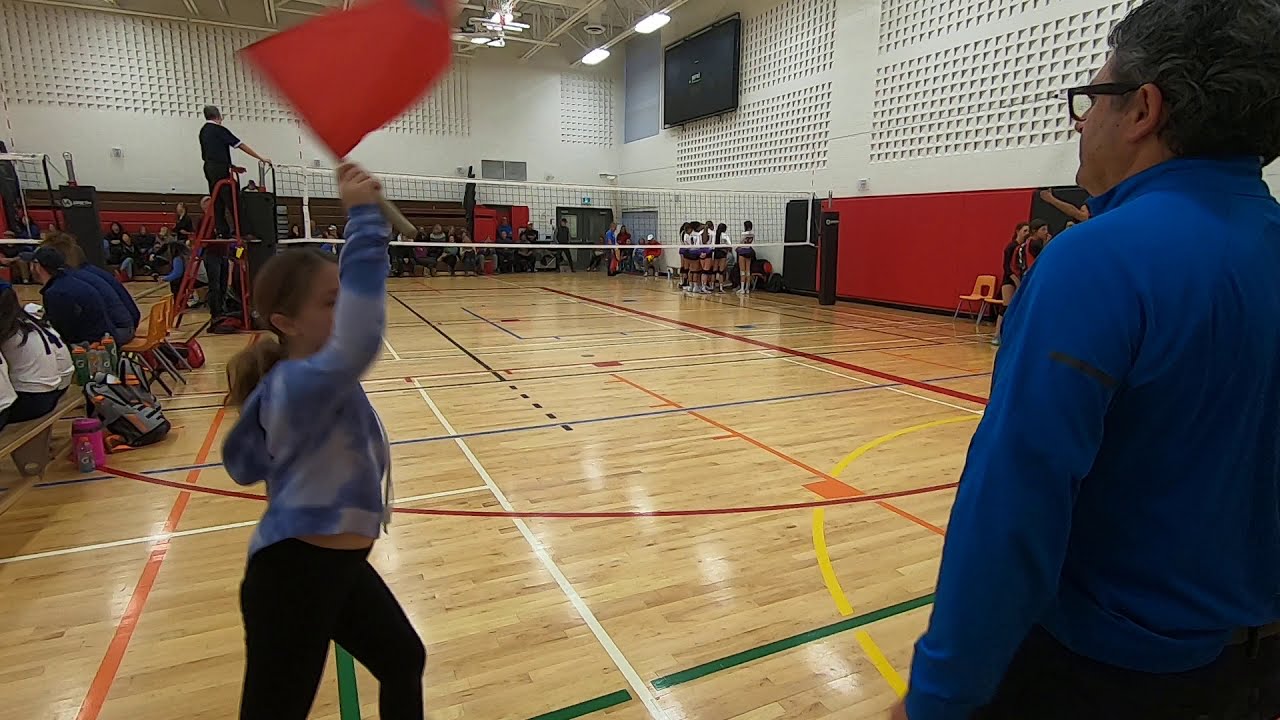In this detailed image, we observe an indoor gymnasium, likely part of a school, hosting a volleyball game. In the bottom right corner, there's an older man with glasses intently watching the match. Next to him stands a little girl waving a reddish-orange flag, suggesting she might be an official responsible for checking if the ball goes out of bounds. The volleyball court is clearly visible, marked by boundaries and a net. A referee stands on an orange metal ladder, overseeing the game to ensure fair play, particularly monitoring any net faults. The background reveals a crowd of fans seated on bleachers, which are half-full, as well as benches occupied by a junior high girls' volleyball team, all appearing to be in their early teens. The color palette of the scene includes various shades of brown, orange, blue, black, green, yellow, and red, adding vibrancy to the setting.